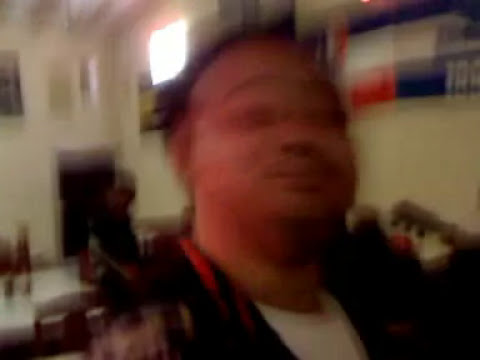In this extremely blurry color photograph, we see a selfie of a slightly overweight man with short dark hair and dark skin, who appears to be around 30 years old. He sports a very thin mustache and is dressed in a white undershirt under a black jacket with white detailing. The photograph, taken indoors in a landscape orientation, portrays the man from his clavicles upwards. Situated behind him over his left shoulder is another indistinct figure, appearing to stand in front of either a doorway or an archway. The room itself features plain white walls and is possibly filled with various household items, including a table and chairs in the bottom left corner. Additionally, a window towards the top left of the image lets in natural light, suggesting it might be daytime. In the background, there’s a red, white, and blue squares banner with unreadable text adding to the details of the setting, which might be a kitchen or another common area inside a home.